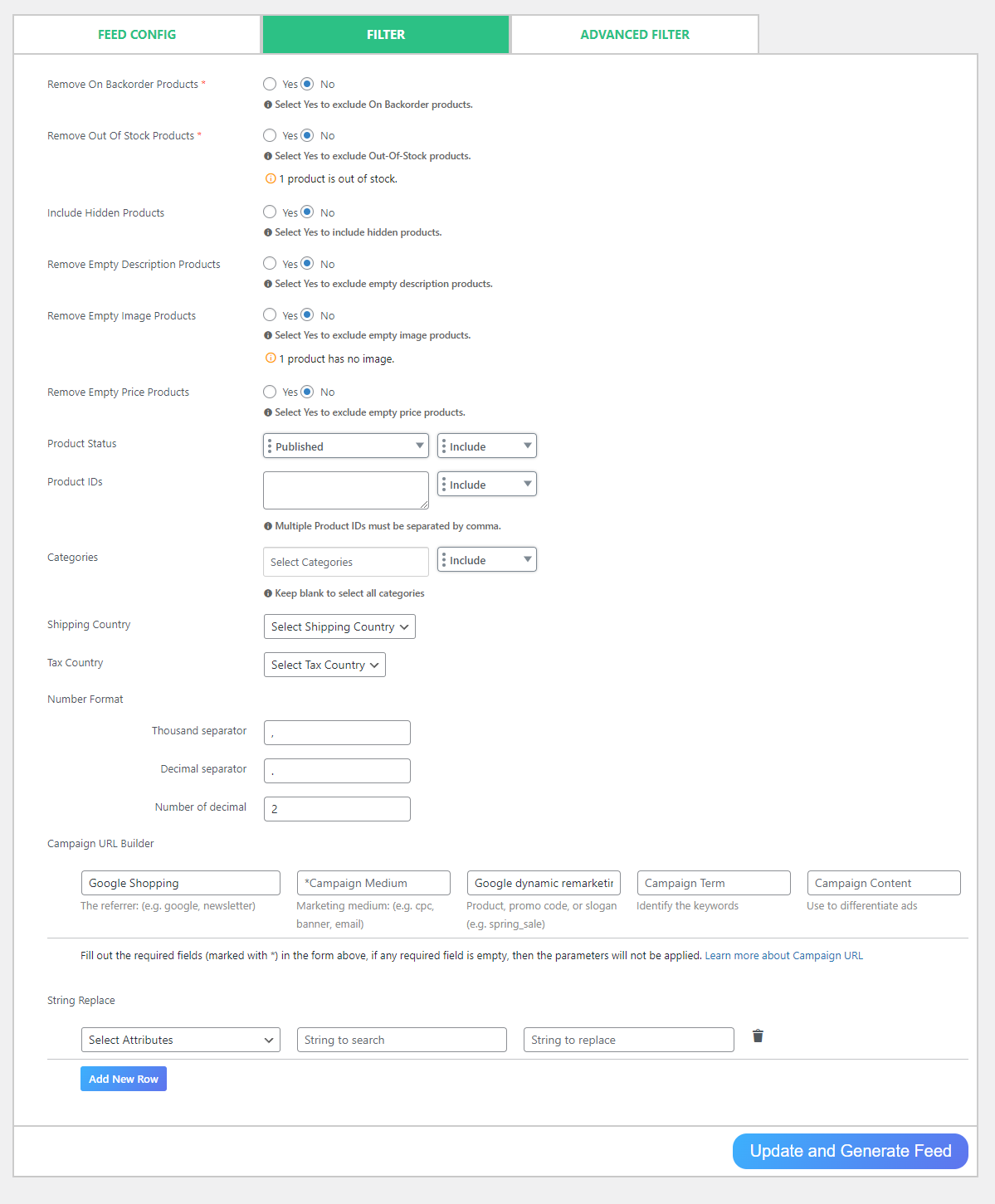The image features a detailed interface displayed on a clean, white background, divided into three tabs at the top: "Feed," "Configure," and "Filter," with the "Filter" tab currently active. The "Filter" tab is highlighted in green with white lettering, while the other two tabs are white with green lettering.

On the left-hand side, several filtering options are presented in a hierarchical format:

1. **Remove on Backorder Products:** 
   - Option to switch between "Yes" and "No"; currently set to "No".
   - A note indicates that selecting "Yes" will exclude products that are on backorder.

2. **Remove Out of Stock Products:**
   - Option to switch between "Yes" and "No"; currently set to "No".
   - A note indicates that selecting "Yes" will exclude products that are out of stock.
   - There is an indication that one product is currently out of stock.

3. **Include Hidden Products:**
   - Option to switch between "Yes" and "No"; currently set to "No".
   - A note indicates that selecting "Yes" will include hidden products.

4. **Remove Empty Description Products:**
   - Option to switch between "Yes" and "No"; currently set to "No".
   - A note indicates that selecting "Yes" will exclude products with empty descriptions.

5. **Remove Empty Image Products:**
   - Option to switch between "Yes" and "No"; currently set to "No".
   - A note indicates that selecting "Yes" will exclude products that lack images.
   - There is an indication that one product has no image.

Below these options are additional settings related to product status and exclusions:

- **Product Status:** 
  - A dropdown menu labeled "Published".
  
- **Exclude:** 
  - A dropdown menu next to "Product Status".

Further down, two empty data fields are available for entry. The first data field appears below "Publish," and the second is below "Exclude." Another note specifies that multiple product IDs must be separated by commas.

Finally, there is a "Categories" section:

- **Categories:** 
  - A data field is available for selecting categories.
  - To the right of this field, a dropdown menu labeled "Include" is present.
  - An additional note suggests using the dropdown to select all categories.

Overall, the interface is filled with various filter options aimed at refining product visibility based on stock status, descriptions, images, and categories.